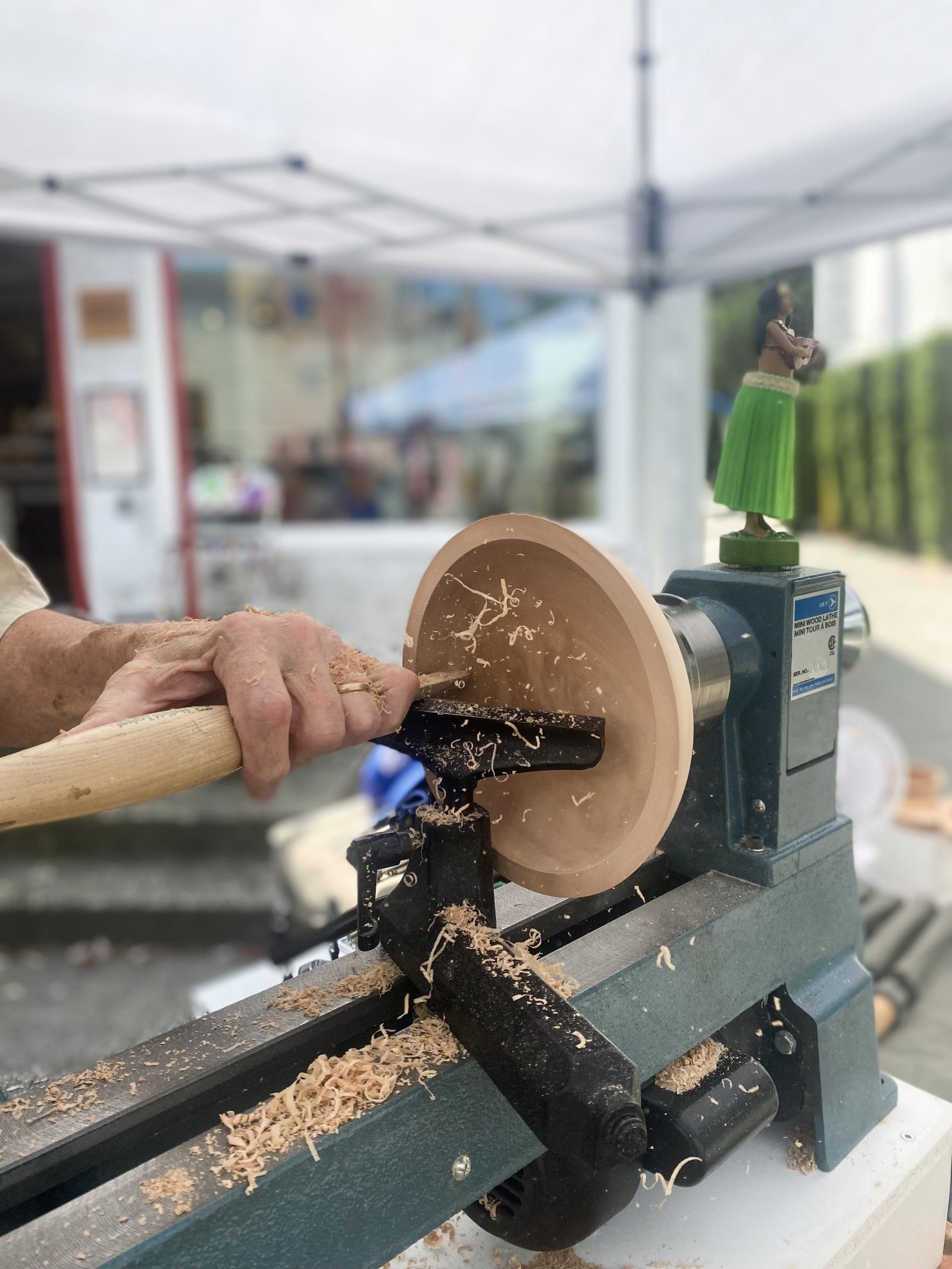This indoor photograph captures a detailed scene of a senior Caucasian man, identified by his leathered hand and gold wedding band, meticulously crafting a wooden bowl. At the center, his hand firmly grips a wooden-handled chisel with a metal tip, intricately shaping and turning a wooden piece on a chisel set. Wood chips and shavings are seen flying through the air, landing below the work area, emphasizing the precision and activity in the scene. A charming, small hula girl figurine, poised to bobble with movement, adds character to the chisel set. The background, though blurry, hints at a well-equipped workshop with various machinery and a window draped with green curtains, suggesting a vibrant, well-lit space perfect for woodworking crafts.